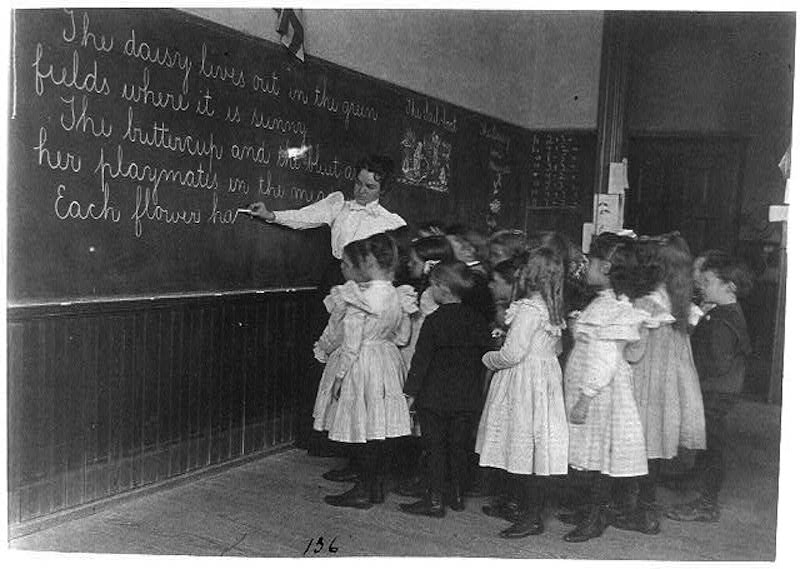This timeless black and white photograph captures an intimate classroom scene from an era long before modern technology, likely predating the 1950s. Taken from a side-view angle, the image features a poised and elegant schoolteacher, adorned in a frilly, lacy outfit with her hair meticulously curled and styled in an updo. She is diligently writing on a chalkboard with cursive text that reads: "The daisy lives out in the green fields where it is sunny. The buttercup and..." though the complete text remains obscured by the crowd of students or veiled in mystery due to the image quality.

The classroom is filled with approximately 15-20 young pupils, both male and female, all attentively focused on their teacher. These children are dressed in what appears to be formal school uniforms reminiscent of their Sunday best; the girls don white dresses, while the boys are clad in black suits, all complemented by dark boots. Notably, instead of sitting at desks, they are standing or hunched together closely in front of the chalkboard, adding a sense of engagement and intensity to the scene.

Details in the background, such as a door and simple wood paneling beneath the chalkboard, complete the old-fashioned classroom setting. At the very bottom of the picture, the numbers "1, 3, 6" can be discerned, though their significance is unclear. The timeless quality of this photograph offers a glimpse into the educational practices and sartorial elegance of a bygone era, capturing a moment frozen in time.